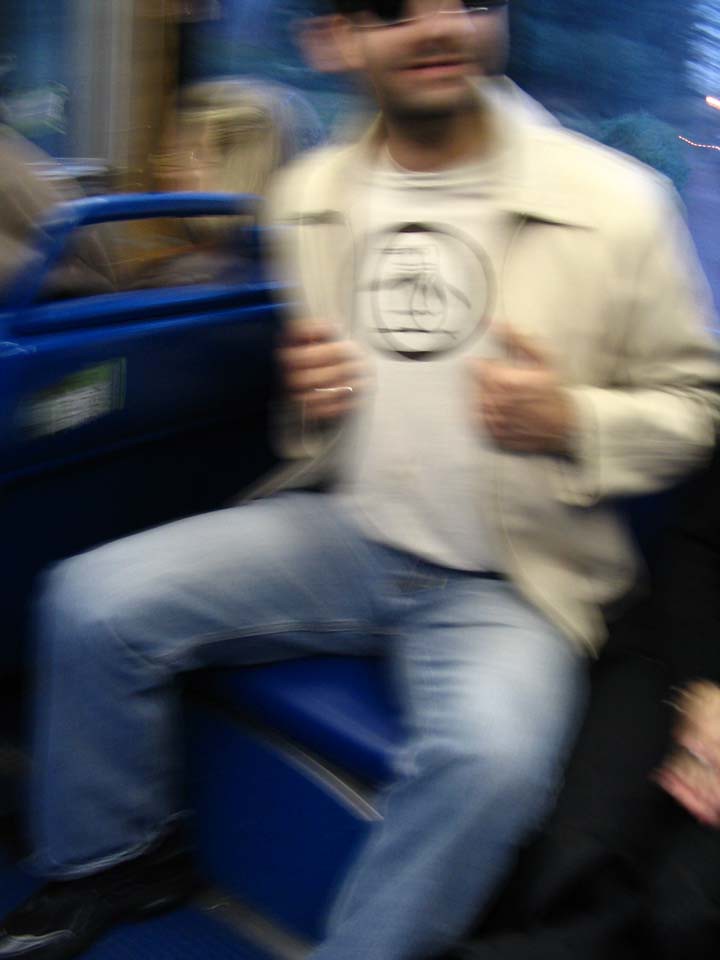The image depicts a slightly blurry scene of a man sitting on a blue chair, possibly on public transportation. He is dressed in an off-white jacket featuring a wide collar and a zipper, underneath which he wears a white t-shirt adorned with a black circular logo that might depict a bird or another symbol. His outfit is completed with blue denim jeans and black shoes. The man has some facial hair, including stubble and a mustache, and is wearing sunglasses. He appears to be holding his jacket open with both hands, possibly to show the logo on his t-shirt. To his right, a blue bench-like structure or a rail can be seen, along with two people sitting perpendicular to him, one of whom has blonde hair with brown roots. The background reveals trees and suggests that the image may have been taken on a bus or train. A black, indistinct object, perhaps another jacket, is visible to the man's left.